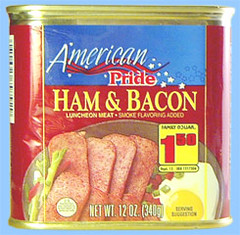The image depicts a rectangular, rounded-corner can of 'American Pride Ham and Bacon' luncheon meat, featuring smoke flavoring. The can has a vibrant design with a blue upper section displaying 'American' in white text and a red lower section with 'Pride' in red text. Below, 'Ham and Bacon Luncheon Meat, Smoke Flavoring Added' is written in yellow. The front showcases an appealing serving suggestion: neatly sliced pieces of ham and bacon beside a sunny side up egg on a plate. A yellow circle highlights the suggested price of $1.50 in red text. Additional details include a barcode peek at the top left and the net weight specification—12 ounces (340 grams)—in small white text at the bottom. The overall background of the can maintains a red theme.